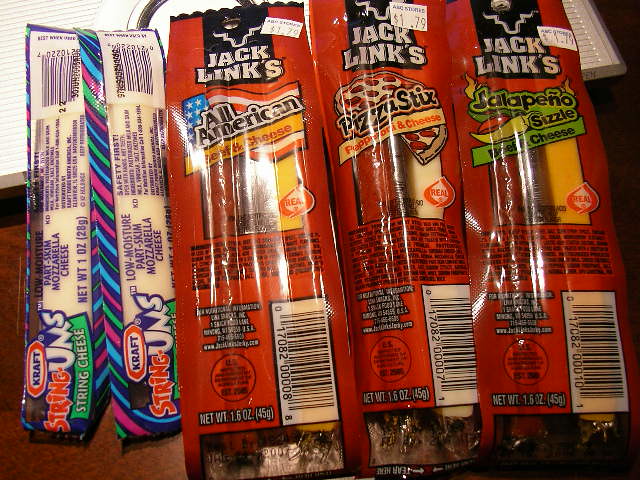This horizontal photograph features a collection of packaged snacks, meticulously laid out side-by-side on a brown countertop with a metallic object underneath them. On the left, there are two Kraft String Ums, labeled as Low Moisture Part Skim Mozzarella Cheese. The packaging is primarily red and white, with a green rectangle and blue writing indicating the net weight of one ounce. The tops of these packages are open, revealing the cheese inside. To the right, there are three packages of Jack Link's beef and cheese sticks, each marked with a price tag of $1.79. The packaging is predominantly red with black accents and a clear window to display the contents. The Jack Link's varieties include All-American Flavor on the far left, Pizza Sticks with pepperoni and cheese in the center, and Jalapeno Sizzle beef and cheese on the right.